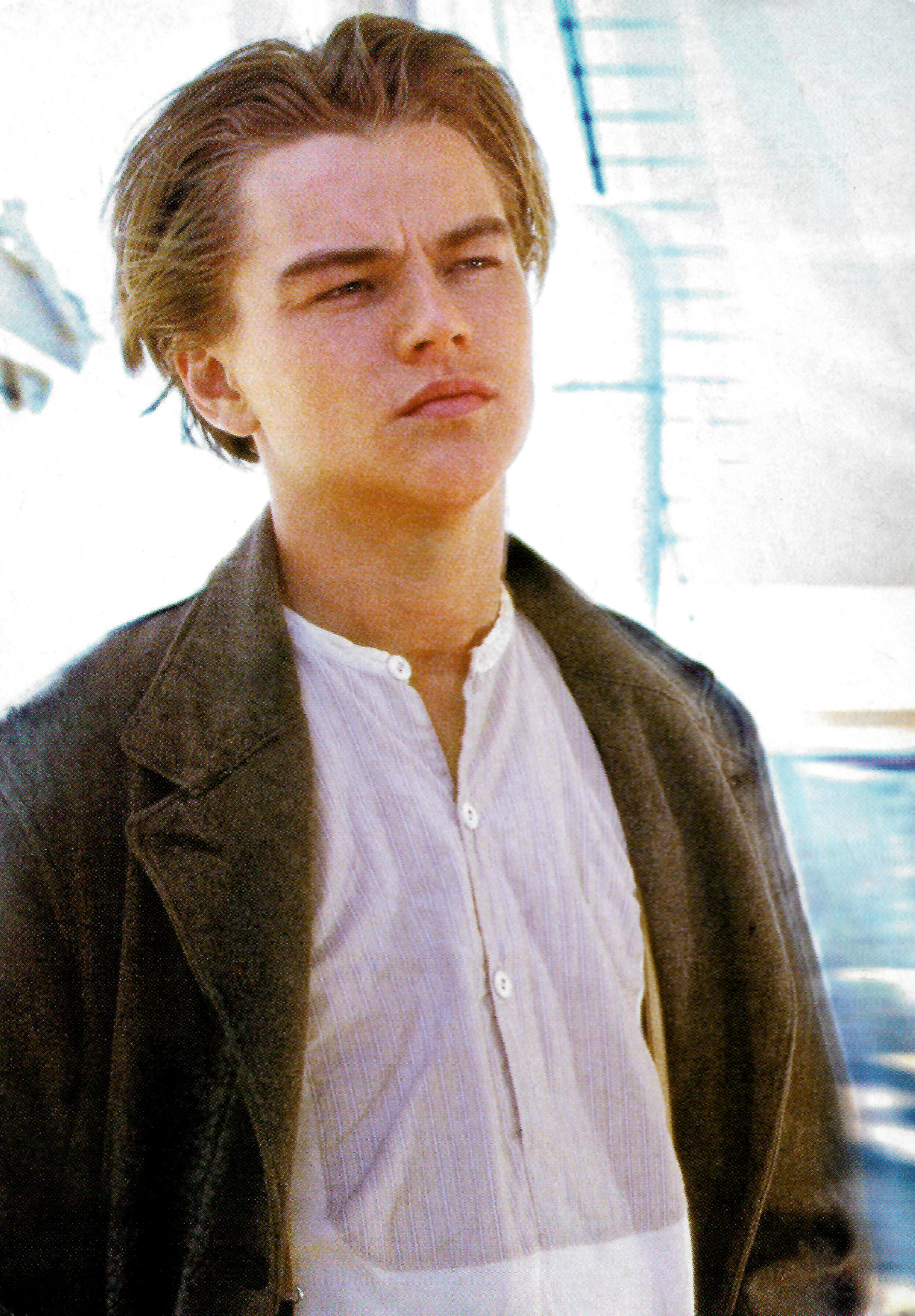The photograph captures a young man dressed in an open brown cloth jacket over a light white t-shirt with three buttons, the top one being unbuttoned. His blonde hair is swept back, giving him a windswept look. Positioned centrally in the image, he gazes to the right with a contemplative expression. The backdrop, though blurred, reveals a large body of clear blue water in the bottom right, contrasting against white, slightly out-of-focus seating below and a white sail or canopy in the upper half. The overall setting appears to be outdoors on a bright, sunny day, creating a vibrant and airy ambiance.